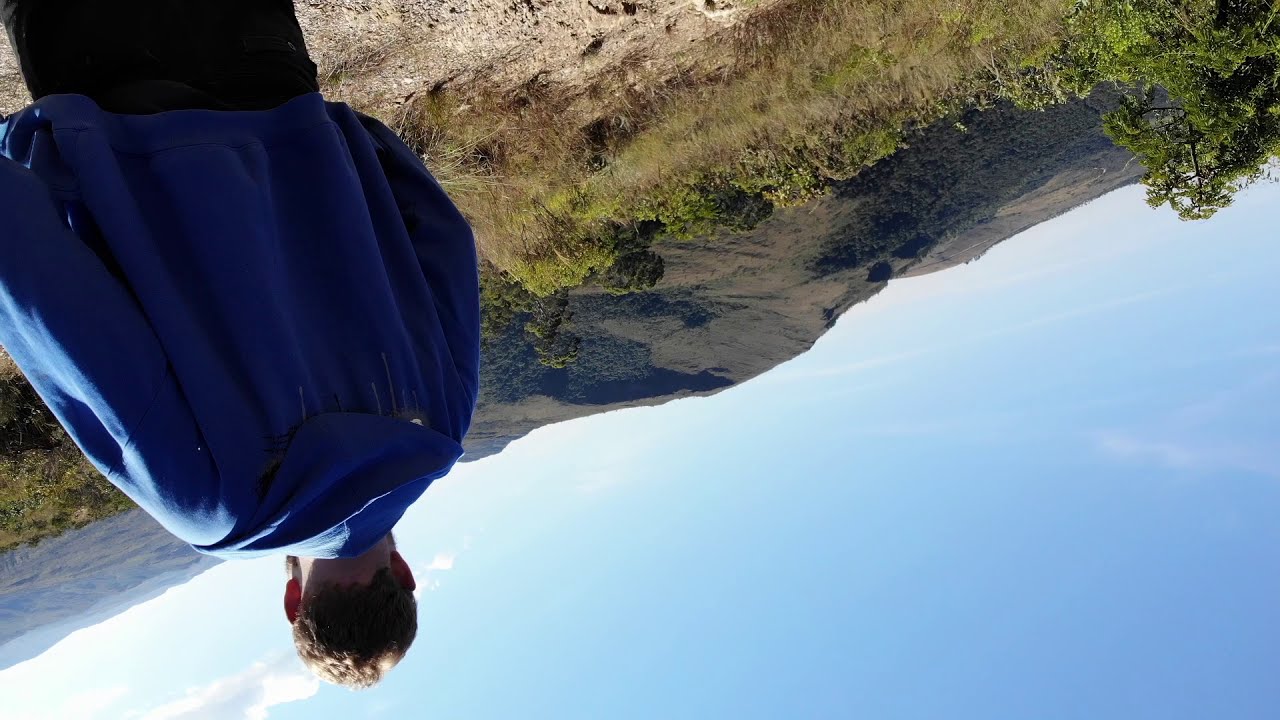In this upside-down, outdoor daylight photograph, a boy with short curly brown hair, wearing a blue jacket and black pants, walks away from the camera. His figure, located towards the top left, is inverted due to the flipped nature of the image. The scene captures a rugged natural landscape, with brown dirt and scattered green shrubs at the top of the image, transitioning to a distant mountain range that appears dark green and rocky, possibly with pathways etched into them. The mountains give way to a bright, blue sky with a few wispy clouds occupying the bottom right of the photograph. A tree also stands inverted towards the top right, contributing to the serene yet disorienting composition of this inverted scene.